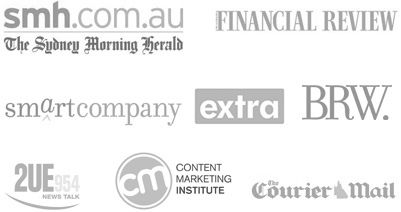The image showcases various news media outlets, each represented by a translucent, light gray label against a white background. The featured media outlets include "Financial Review," "Extra," "BRW," "Smart Company," "Content Marketing Institute (CM)," "The Courier Mail," and "The Sydney Morning Herald," with its website noted as smh.com.au. In total, there are eight different news media companies presented. The light gray, almost see-through appearance of the labels gives them a subtle, faded look, blending slightly with the background. The overall effect is a minimalist and ethereal collage of media brand names.